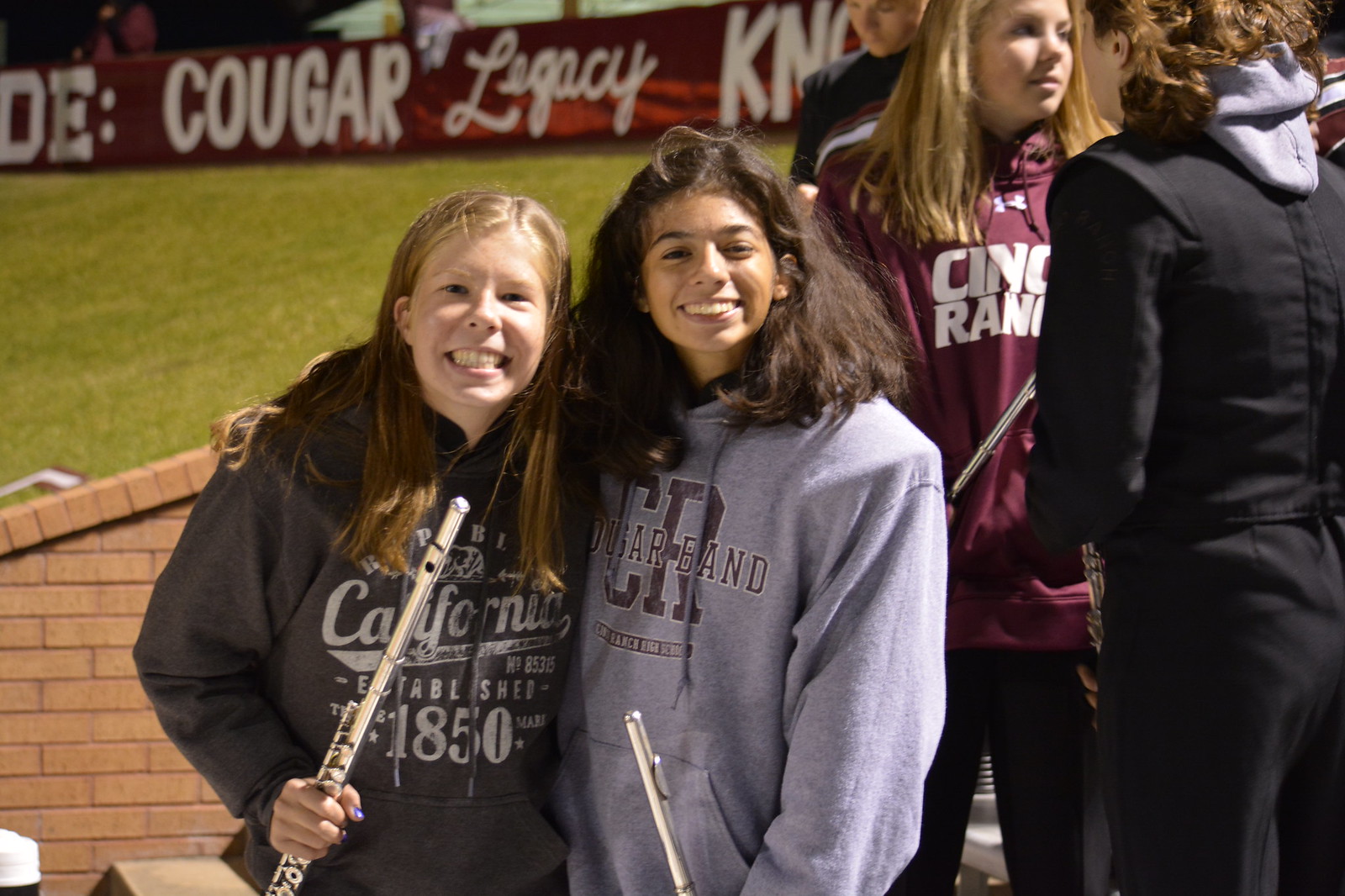This outdoor photograph captures two teenage girls standing side by side and hugging, with big smiles on their faces as they pose for the camera. They both have long hair; the girl on the left sports light reddish-brown hair while the girl on the right has thick, frizzy dark brown hair. The girl on the left is wearing a dark hoodie with "California Established 1850" written on it, while the girl on the right dons a gray hoodie. Both girls are holding flutes. They appear to be on the edge of a sporting field, and behind them, there are more girls congregating. One has blonde hair and looks to be around 18 years old, while another girl facing her is dressed in all black with a gray hoodie, also holding a musical instrument. In the background, a red banner with white text reads “Cougar Legacy.” The scene suggests a setting such as a practice field or stadium bleachers, with a brick wall and grass visible behind the group.